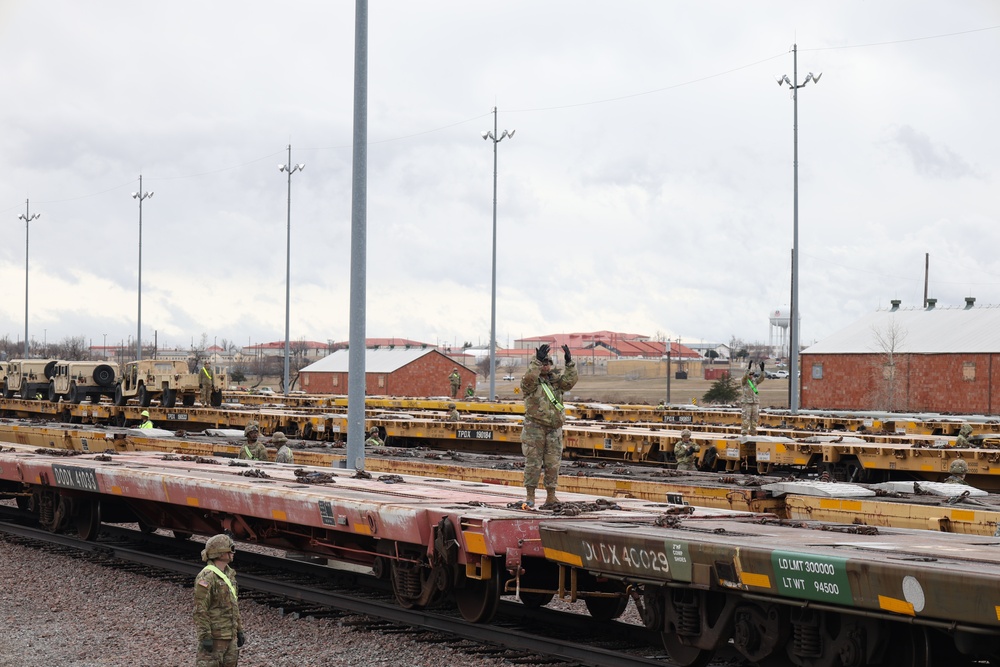This photograph captures a bustling scene at a railway station under a gray, cloudy sky, suggesting a cold climate based on the thick attire of the people present. The station appears to function as a military depot, evident from the numerous flat, empty train car beds lined up along the tracks, waiting for cargo. Prominently, two military members in green camouflage uniforms are actively involved in directing operations; one stands by the train tracks while the other is perched on a train car bed, both gesturing to coordinate the loading process. In the background, military Hummers are clearly visible atop one of the train beds, reinforcing the notion that this facility is used for transporting heavy military equipment. Additional personnel are scattered around, contributing to the logistical efforts. Despite the overcast conditions, the photograph provides a vivid glimpse into this rarely-seen aspect of military logistics.